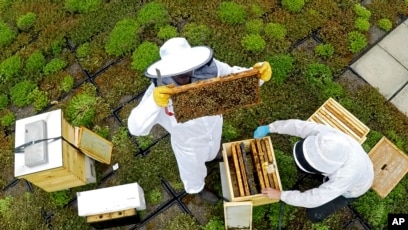In this photo, we see two beekeepers fully dressed in their protective white suits, including netted masks, and gloves. One beekeeper wears yellow gloves, while the other wears a blue glove on their right hand and has no glove on their left. They are meticulously inspecting the beehives; the standing beekeeper is holding up a honeycomb tray teeming with bees, examining it closely, while the kneeling beekeeper appears to be retrieving another tray from an open hive. Surrounding them are several other beehives—around five in total—and various boxes and lids scattered about. The background is lush and green with various plants growing, indicating that they are outside. The scene is bathed in daylight, and a concrete surface is visible behind them. Despite the activity, no bees are seen flying around in the immediate vicinity.